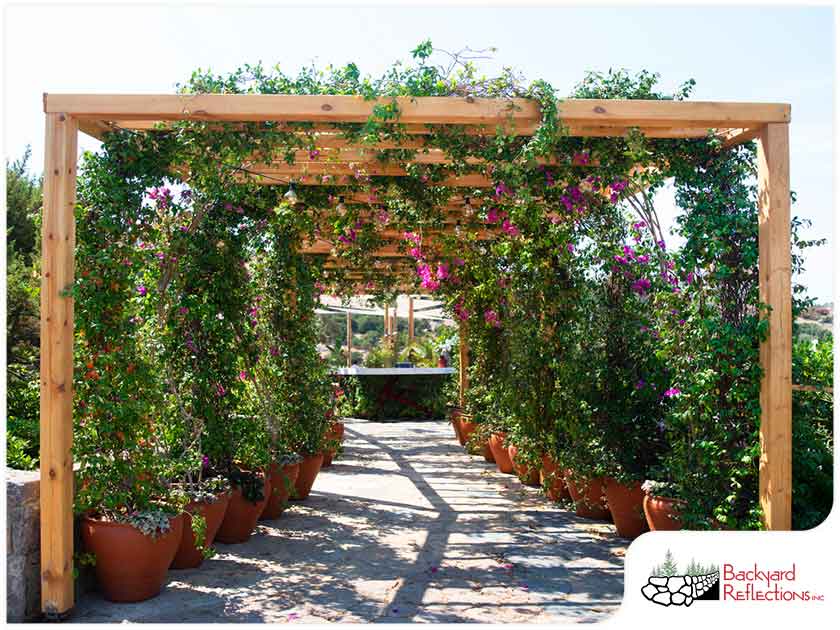The photograph depicts a vibrant outdoor scene at what appears to be a garden nursery or a garden architectural shop. The focal point is a large wooden trellis, made of cedarwood, with a series of horizontal and vertical posts creating a structured framework. This trellis is adorned with a variety of vines and plants, many of which have pinkish-purple flowers, cascading over the top and sides. The plants are growing from various pewter and terracotta pots that line the gravel pathway running through the center of the image.

In the background, more greenery and a bright blue sky are visible, enhancing the outdoor ambiance. The bottom right corner of the photo features a small, intricate black-and-white sketch of a stone wall with green trees behind it. To the right of the drawing, the text "Backyard Reflections, Inc." is prominently displayed in red letters. This blend of natural elements and artistic touches offers a detailed and picturesque view of the garden setting.